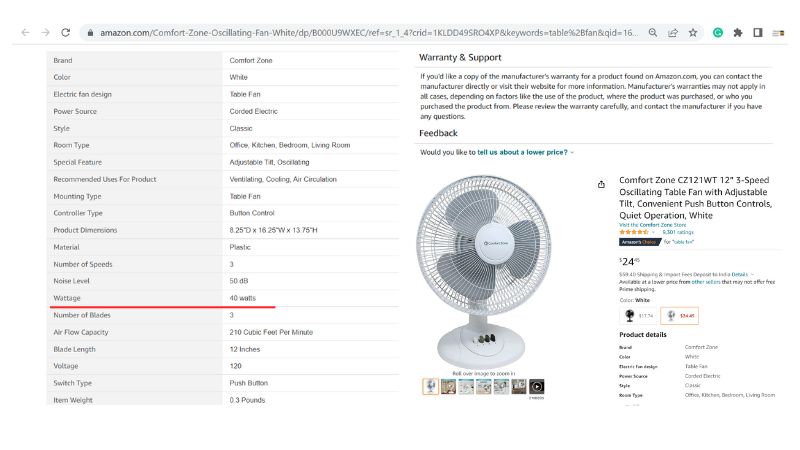The image primarily features an intricate user interface layout or product listing, rich in graphical elements and text details.

---

On the upper left-hand side of the image, there are navigation arrows pointing left and right, adjacent to a circular icon with an embedded arrow. A grey bar featuring a lock icon and what appears to be a URL is situated next to a magnifying glass icon. To the right of this set, an assortment of symbols can be seen: a curved arrow pointing right, a star, a green-blue circle with a white segment, and a couple of indistinct black symbols. Additionally, two rectangles (one white with a grey outline and one grey attached to it) are discernible, followed by a light grey dot and a dark purplish-grey dot. The text surrounding these elements is too small to read.

Further down the image, a light grey rectangle on the left-hand side contains text, peaking out prominently at about three-quarters of the way down. Here, a striking red line extends beyond the rectangle, leading into a white section populated with various unreadable words. Central to this lower section is the image of a fan, beneath which sit additional, smaller and indistinct images.

On the right side of the image, detailed product information reads: "Comfort Zone, CZ121WT, 12-inch, 3-speed, oscillating table fan with adjustable tilt, convenient push-button control, quiet operation white." Underneath this description is a series of blue words, followed by a line of yellow stars indicative of a rating system, and a unique, black slanted rectangle on the right side marked with "24" and some additional text that is too small to decipher.

---

The composition of the image indicates a detailed product listing page, possibly from an online store, replete with navigational, interactive, and descriptive components.